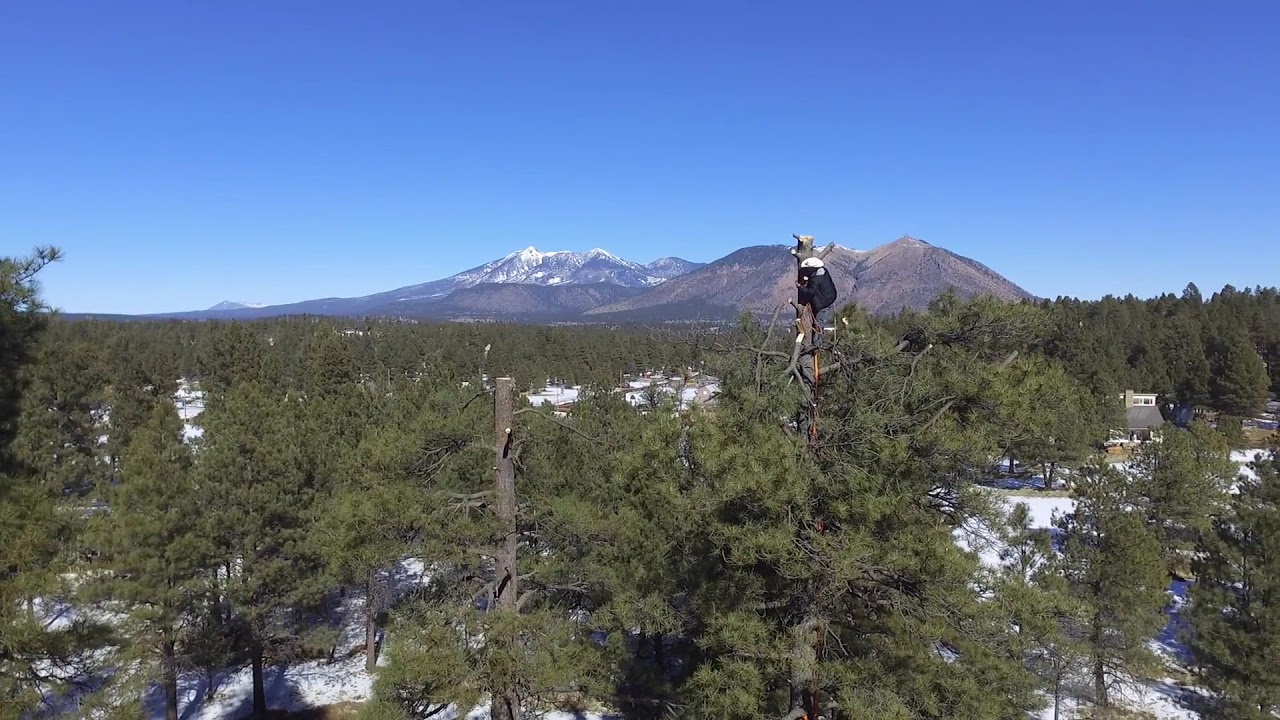The image captures a logging scene set against a breathtaking mountain landscape. In the foreground, a logger, identifiable by his white helmet and long-sleeved black jacket, is perched high on a pine tree, using orange ropes for support. He is in the process of cutting the top off the tree. Nearby, another tree has already been topped to a similar height. This scene is observed from an elevated vantage point, possibly from a drone or another tree. The background features a series of majestic snow-capped mountain peaks under a gradient blue sky. The ground below is blanketed in snow, interspersed with orderly rows of pine trees, suggesting a tree farm. Some trees are markedly shorter, indicative of recent logging activities. Among this wintry wilderness, a small, barely visible house with a gray roof and chimney peeks out through the trees on the right. Additionally, a tall tree near the central activity has a black bag or object hanging from it, adding an element of mystery to the rugged, yet serene, mountain environment.